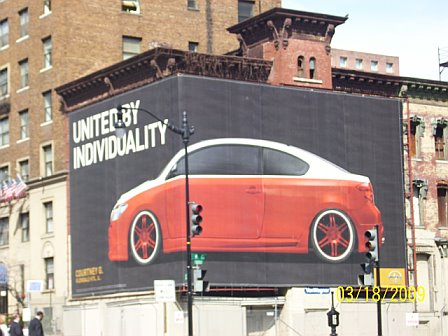This image captures the vibrant side of a building in an urban area characterized by multiple brick apartment buildings. Prominent in the scene are stoplights, hinting at the bustling nature of the location. The focal point of the photograph is a striking mural that adorns the side of the building. This mural, set against a black backdrop, features an orange car and is emblazoned with the slogan "United by Individuality" in bold white letters, suggesting it is a car advertisement. While the car's make and model aren't distinguishable due to the image quality, there is additional text to the left of the mural that appears blurry. The photograph itself seems dated, with a timestamp indicating it was taken on March 18th, 2009.